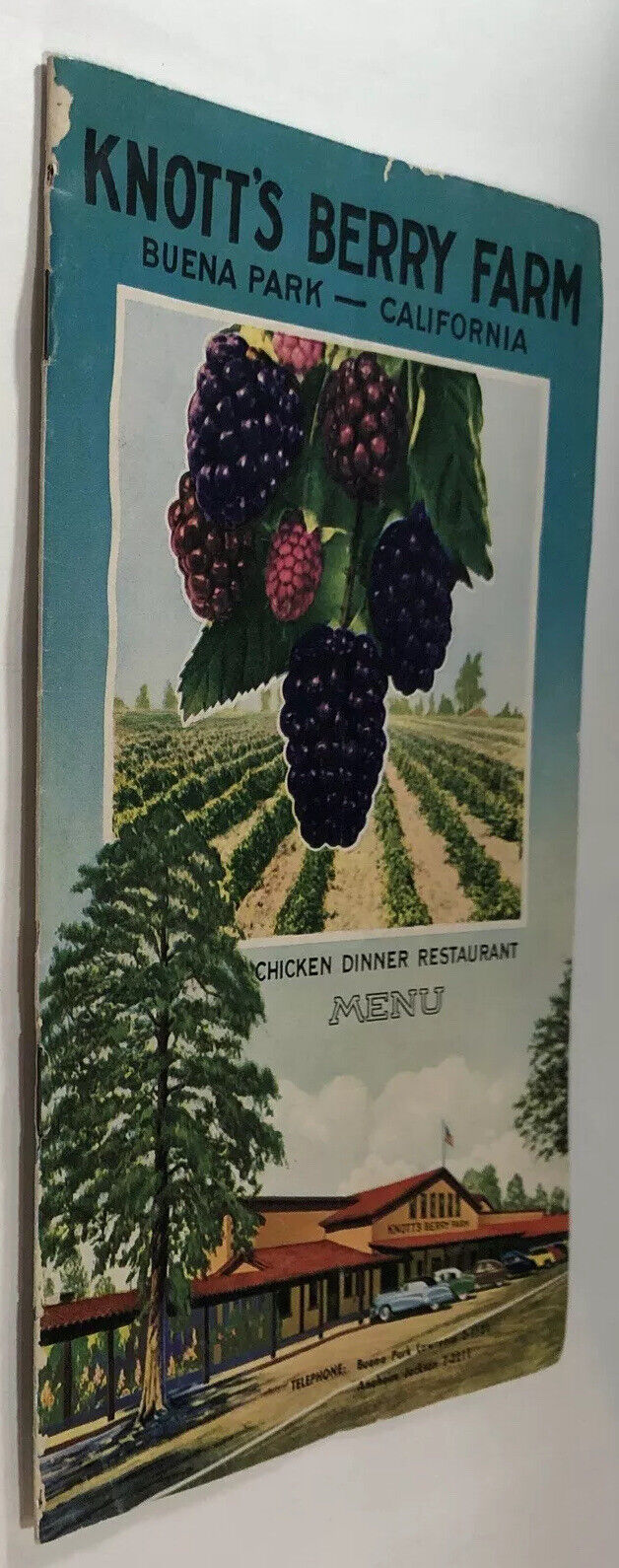This image displays a vintage and worn pamphlet for Knott's Berry Farm, situated in Buena Park, California. The pamphlet, possibly laid on a table or viewed at an angle as if hanging on a wall, captures a nostalgic advertisement for the historic Chicken Dinner Restaurant. At the top, prominent text declares "Knott's Berry Farm," followed by "Buena Park, California." Below this header is an image of blackberries, still on the vine, set against rows of plants in a field. The background features a clear blue sky, enhancing the rustic charm of the presentation.

Central to the pamphlet is the bold inscription, "Chicken Dinner Restaurant Menu." An artistic illustration beneath this text portrays the restaurant with a distinctive red roof and orange terracotta walls, adjacent to a large tree on the left. The scene includes detailed renderings of parked cars and surrounding greenery, giving a glimpse of the establishment's bustling atmosphere. Despite the wear along the edges, this pamphlet remains a cherished piece of Americana, highlighting a beloved dining spot at Knott's Berry Farm.